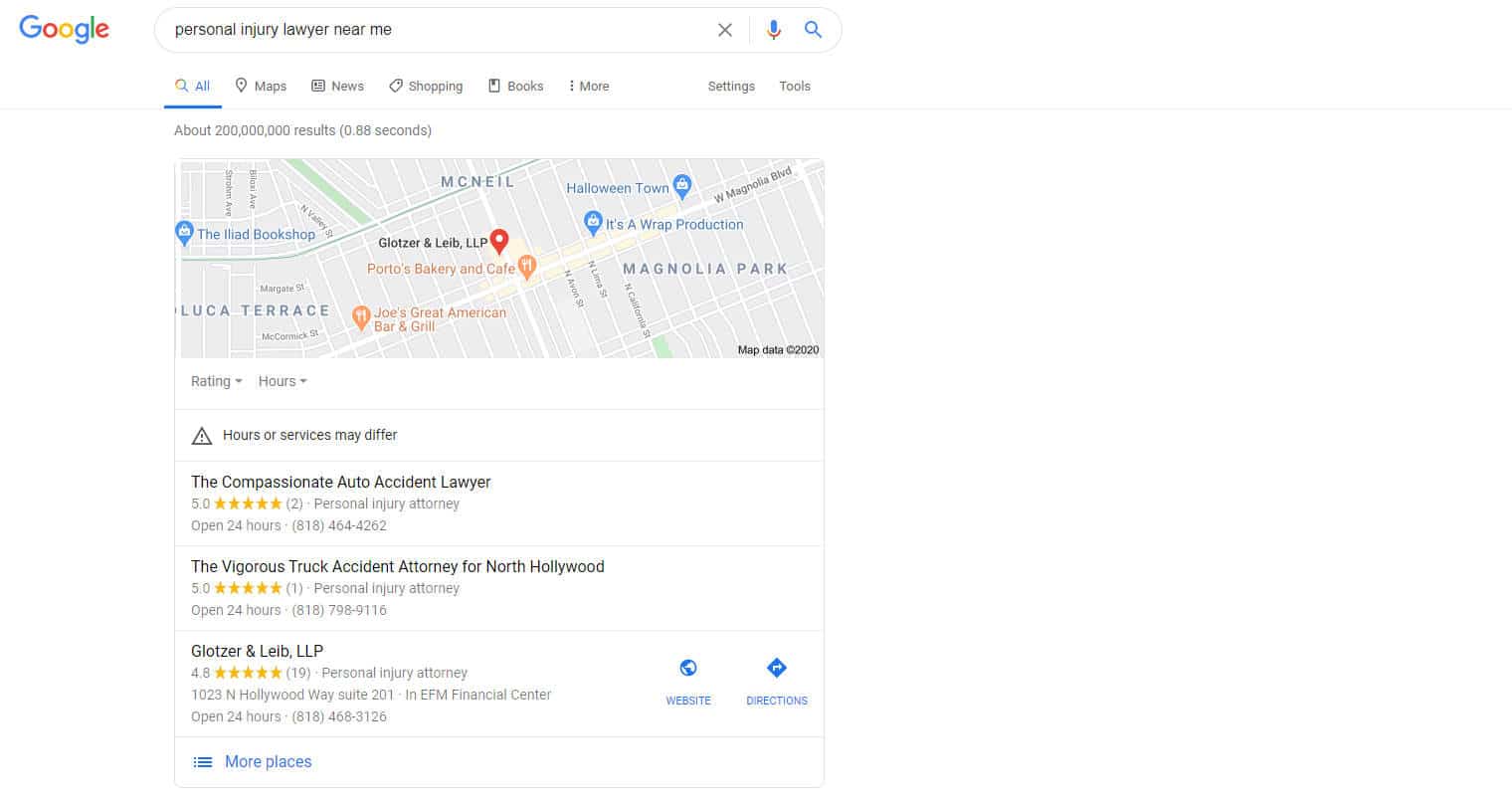A detailed Google search results page for "personal injury lawyer near me" is displayed. The main search bar at the top includes a microphone icon for voice input, a magnifying glass icon for text search, and an option to exit the search. The page is currently in blue highlight mode.

Below the search bar, there are tabs for Maps, News, Shopping, Books, More, Settings, and Tools. The search yielded approximately 200 million results in 0.88 seconds. Directly beneath this information is a Google map featuring various pins that mark relevant locations. Highlighted areas include McNeil Region, Magnolia Park, and the partially visible Luca Terrace. Different attractions and businesses are marked with blue pins, such as E-Lit Bookshop, It's a Wrap Production, and Halloween Town. A red pin indicates Gloucester and Live, LLB, while orange utensils mark food establishments along with their names.

The map data is from 2020. Underneath the map, there are listings for three different personal injury attorneys. Above these listings, a disclaimer states, "Hours of service may vary."

1. **Compassionate Auto Accident Lawyer**
   - Rating: 5 out of 5 (based on two reviews)
   - Contact Information: Includes open hours and a phone number.

2. **Bigger Truck Accident Attorney**
   - No additional details provided in the description.

3. **Gloucester and Live**
   - This entry includes a website link, depicted by a globe icon, and directions to the location.

There are also options to view more places further down the list.